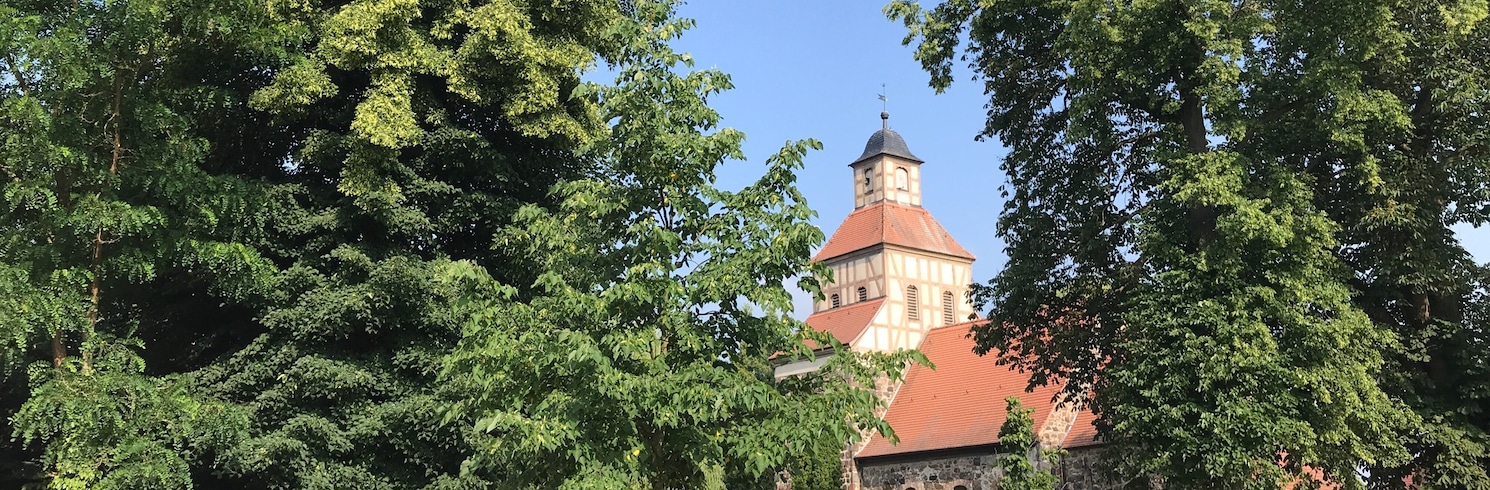The photograph captures a serene forest setting with a densely packed array of thick trees, predominantly showcasing various shades of green. These trees are so close together that visibility through them is minimal. Positioned centrally towards the bottom of the image, the photograph reveals a church in the midst of this lush greenery. The church, characterized by its distinctive steeple, has an orange terracotta-tiled roof, white walls accented with wooden beams, and brown stripes. The steeple, topped with a gray roof resembling that of a bell tower, is visible above the structures below. The church's walls transition to brickwork near the base where the trees obscure further details. The image's palette includes greens from the foliage, reds from the roof tiles, whites and grays from the church structure, and the light blue expanse of the sky visible through a break in the trees. The composition captures the church nestled among evergreen trees, creating a peaceful and secluded woodland scene.